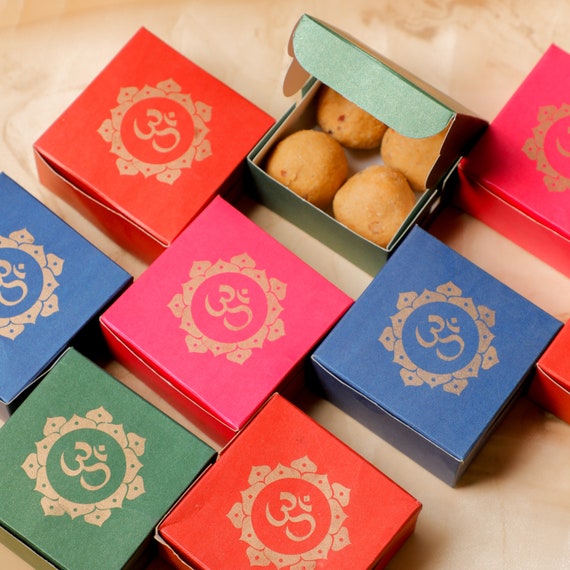The image depicts an assortment of five closed boxes and one open box, all resting on a table covered with a tablecloth. The closed boxes are arranged in the bottom half of the image, while the open box is centered towards the top. The boxes are in various colors, including red, pink, light blue, green, and tan, and feature cursive text displaying the number "30" on their tops. The open box reveals four golden-brown muffins arranged in a 2x2 grid. Despite the different interpretations of the contents, the consensus is that they are muffins. The setting appears to be a simple, staged display to showcase the colorful boxes and their baked contents.